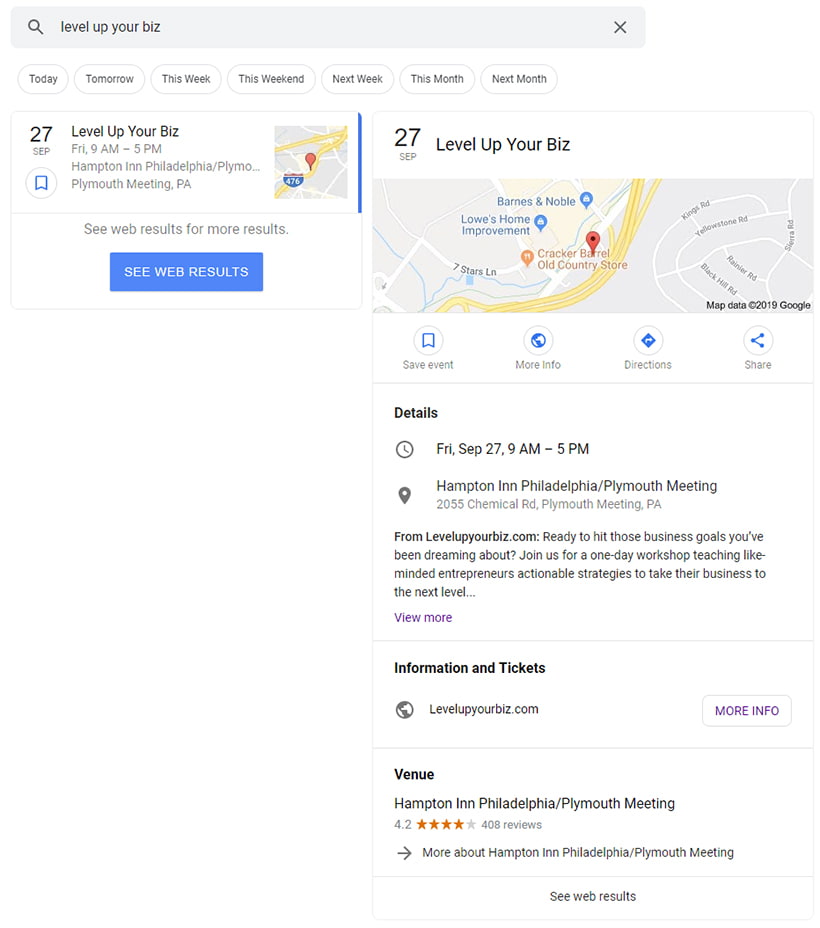The image displays a travel-oriented website layout. It features a structured layout designed to assist users in exploring and planning events. 

- In the upper left-hand corner, there is a gray banner, which includes a magnifying glass icon. Next to this icon, the phrase "Level Up Your Biz" is prominently displayed. To the right-hand side of this banner, there is an 'X' icon.

- Below the banner, there are oval-shaped tabs with white backgrounds labeled as follows: "Today," "Tomorrow," "This Week," "This Weekend," "Next Week," "This Month," "Next Month."

- Directly beneath these tabs, the text "Level Up Your Biz" is repeated. To the left, the date "27 SEP" is enclosed in a small circle featuring a bookmark icon.

- Below "Level Up Your Biz," the event details specify: "Friday, 9 AM to 5 PM," albeit partially cut off, and the location "Plymouth Meeting, PA." A map icon is also present here.

- A blue rectangle labeled "See Web Results" appears farther down the page, followed by the text, "September 7th, Level Up Your Biz." This leads to a larger map display.

- Adjacent to the map, there are four icons labeled: "Receive," "More Info," "Directions," and "Share."

- The event’s detailed information follows this, reiterating the date and time as "Friday, September 27th, 9 AM to 5 PM," along with the location.

- A paragraph elaborates on the event, with certain words highlighted. The next section titled "Information and Tickets" includes website details and a "More Info" link.

- Finally, the venue information is provided, stating "Hampton Inn Hotel Plymouth Meeting" with a 4.2-star rating.

The careful structure makes it easy for prospective attendees to find relevant event details and navigation options swiftly.